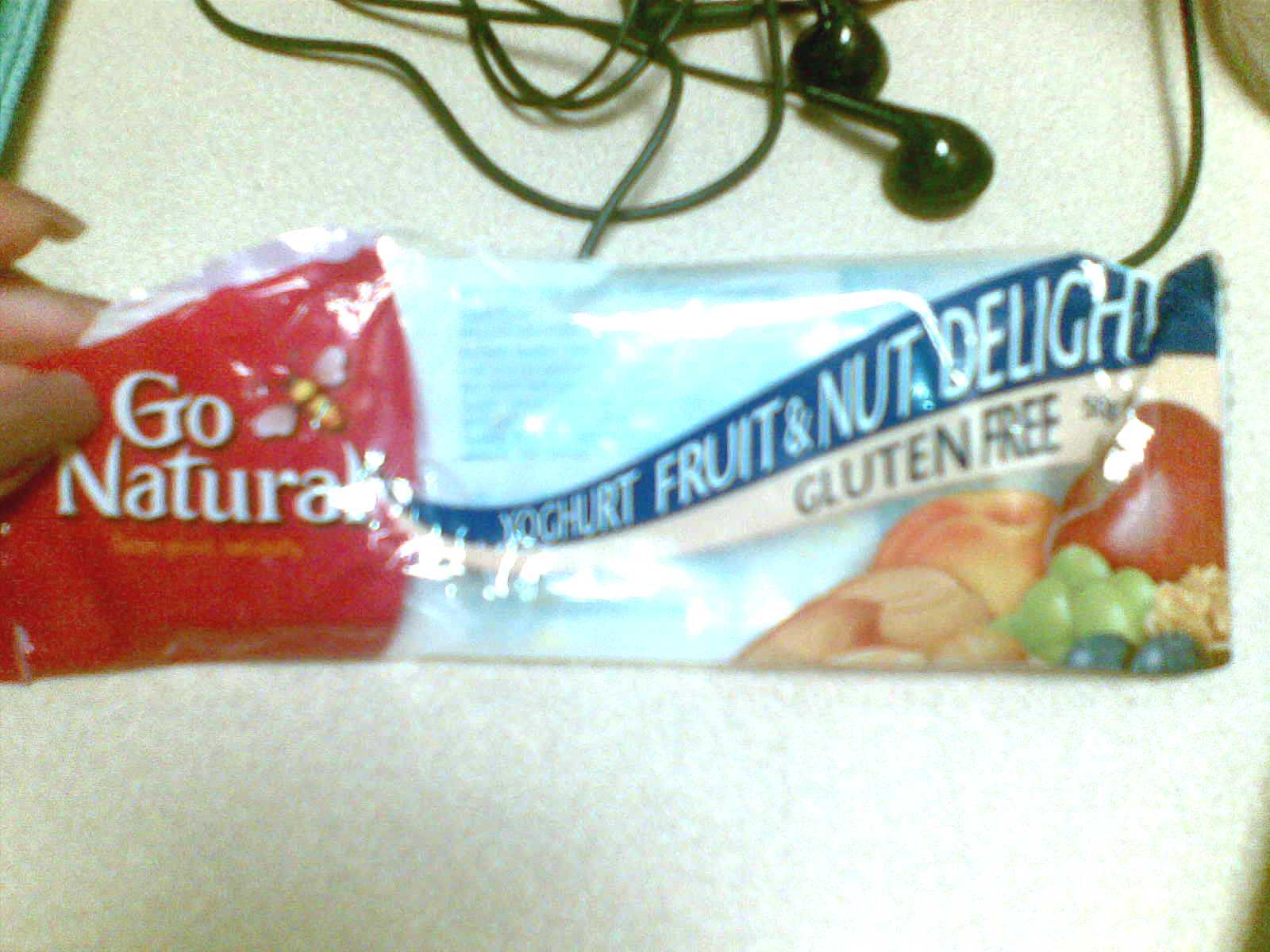A detailed photograph features a hand with long, polished fingernails gripping a package of Go Natural Gluten-Free Yogurt Fruit and Nut Delight. The package displays vibrant images of apples and grapes in the bottom right corner, indicating its contents. Surrounding the package on an off-white surface lies a pair of black vintage corded earbuds, their cords loosely spread out towards the top of the image. The composition suggests a snack break at a desk, combining a nutritious treat with an element of nostalgia through the classic earphones.